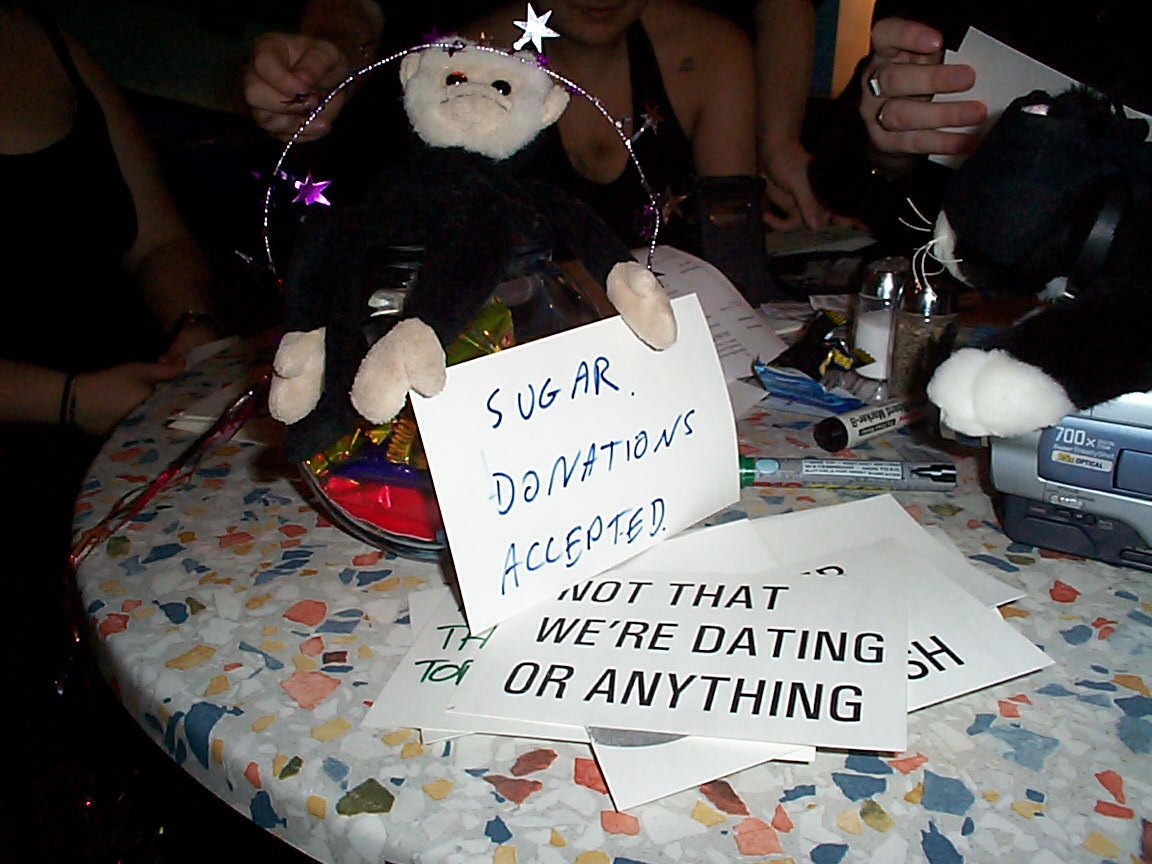In a dimly lit room, the photograph captures a table covered with a stone-colored pattern, featuring a mix of red, blue, yellow, and white fragments. At the center of the table is a handwritten sign in blue pen that reads "Sugar Donations Accepted," propped up by the hands of a cuddly toy monkey. The monkey is positioned inside a ring to the center-left of the image. In front of the monkey lies a printed card displaying the message "Not that we're dating or anything." The cluttered table also holds various markers, some in green and black, along with pens and other miscellaneous items. A fluffy toy cat sits on the right side of the table, near a camcorder. In the background, partial views of people, dressed in dark clothing, are visible, seated around the table, their faces not in the frame but with some arms and the tops of their figures discernible. The room is otherwise dark, with illumination primarily focused on the table.